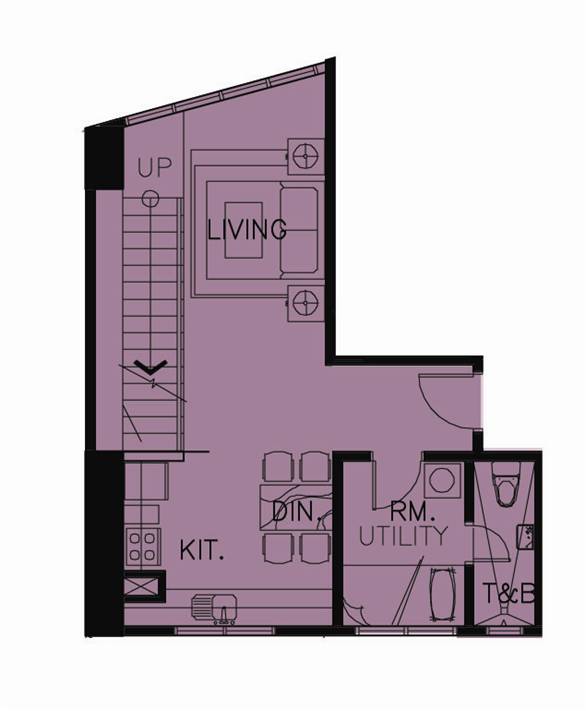This color architectural drawing, presented in portrait format, offers a detailed cross-section and bird's eye view of a home's interior layout, enabling a unique perspective through the ceiling. The image highlights the building’s dimensions and the boundaries that define various sections of the facility. The interior spaces are predominantly illustrated in purple, while the exterior walls and some interior partitions are depicted in black.

The primary area showcased is the living room, identifiable by a couch oriented towards an adjacent wall. To the left of the living room is a staircase leading upstairs. However, the upper level is not visible in this particular drawing, as indicated by a break line that terminates the representation at the stair's ascent.

Adjoining the living room is an open-plan kitchen, seamlessly extending into a dining area furnished with a table and two chairs on each side. Additionally, the drawing includes an RM utility room and a T&B space, denoting a toilet and bath. This intricate depiction provides a comprehensive understanding of the home's functional zones and spatial organization.